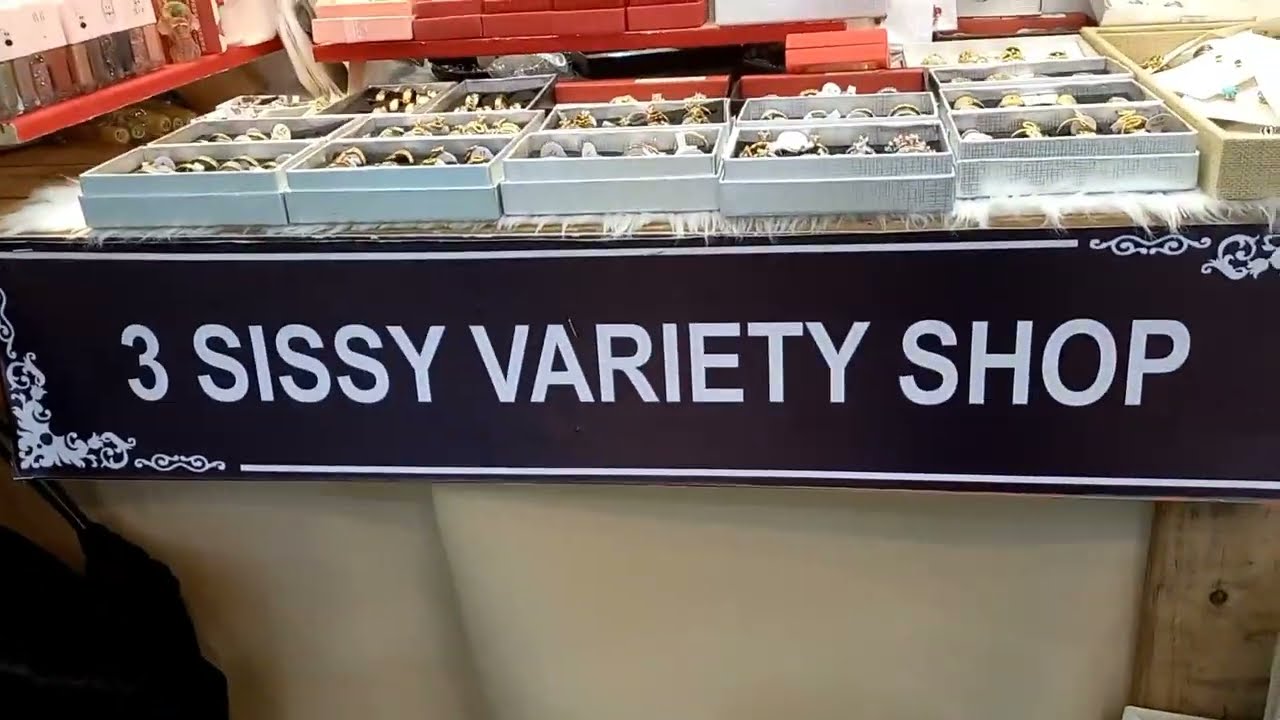The image shows a detailed display of various jewelry pieces showcased on a wooden stand covered with a furry tablecloth. Arranged neatly on the stand, there are fifteen open white and silver jewelry boxes, their lids tucked underneath, revealing shiny items like watches, earrings, and large rings. These jewelry pieces are laid on a gray material, making it difficult to discern their exact nature. The stand prominently features a black sign with white borders and ornate patterns in the corners, reading "Three Sissy Variety Shop" in bold white letters. In the background, additional bright red boxes are visible, hinting at a broader colorful display within the shop's bright, well-lit setting.